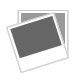The advertisement is set against a white background, featuring bold red text at the top that reads "Mela '88." Beneath that, in slightly smaller red letters, it says "Festival of India." The central illustration showcases three Indian folk dancers dressed in elaborate red and white attire. On the left is a woman adorned in a fancy garment with intricate patterns. She strikes a graceful pose with her right arm raised and her left arm extended outward, wearing a decorative headdress. In the center stands a man, also in red and white, dancing energetically with his feet mid-air and donning a traditional Indian hat. On the right is another woman, similarly dressed with a headdress, her hands and arms lifted high. Her flowing skirt, embellished with triangular patterns, reveals her bare feet. All three dancers display a dynamic and vibrant spirit, with their outfits and movements reflecting traditional Indian cultural elements.